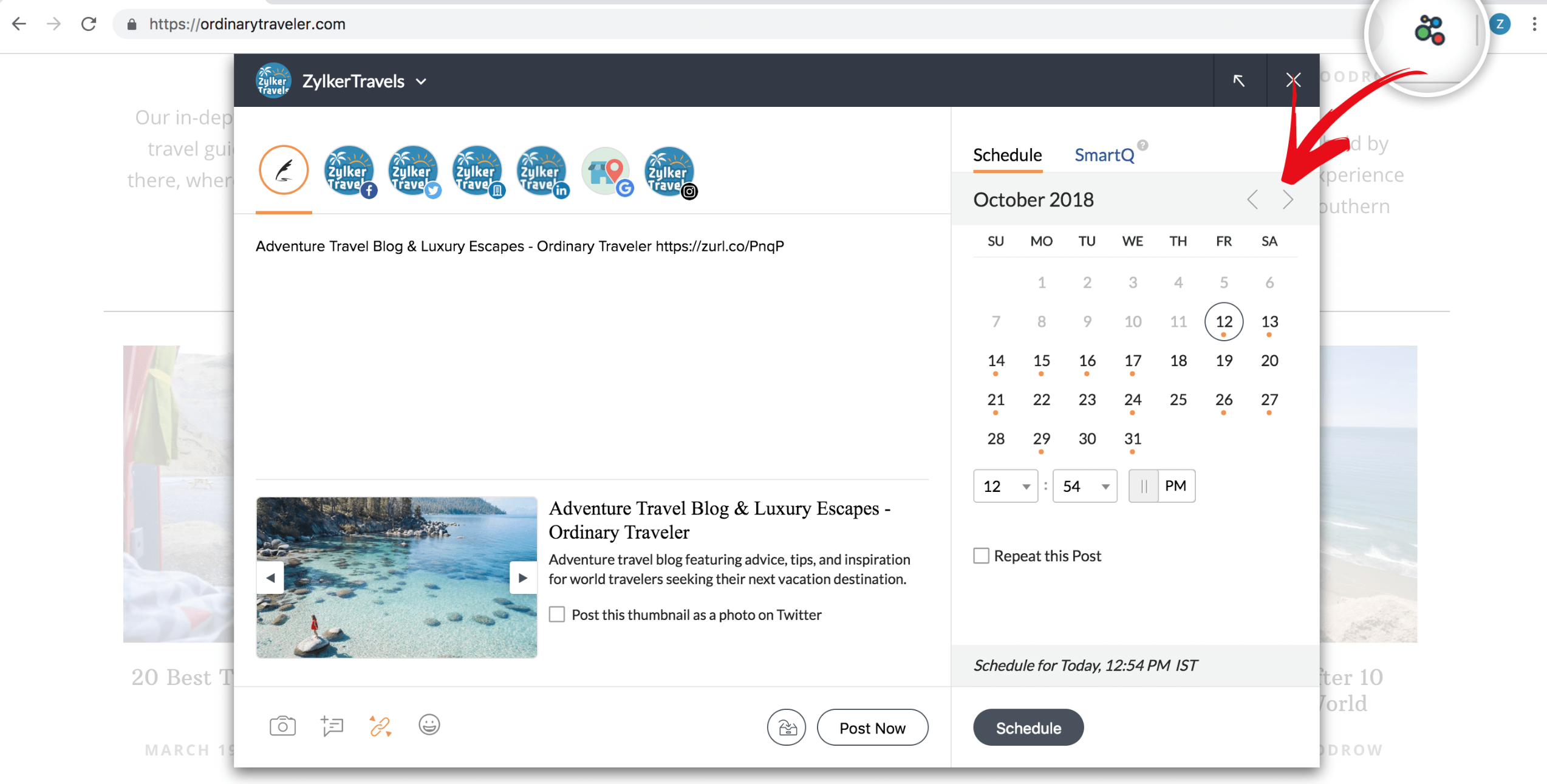The image depicts a webpage from the website ordinarytraveler.com, branded with the title "Xylicor Travels." At the very top of the screen, a prominent black bar runs across, with the name "Xylicor Travels" clearly displayed in white text accompanied by a small blue icon. Below this, several blue icons presumably related to travel categories or services are present.

On the right side of the webpage, there is a section titled "Smart Schedule," indicating a schedule dated October 2018, with a specific time set at 12:54 p.m. Additionally, it mentions an event scheduled for today at the same time. This scheduling information is complemented by a visible calendar displaying the month.

To the left of the schedule, the main content area features a picturesque image of an ocean scene with a person standing on rocks. Adjacent to this photo, on a white background with black text, the title "Adventure Travel Blog and Luxury Escapes: Ordinary Traveler" is prominently displayed. Below the title, a description reads: "Adventure Travel Blog featuring advice, tips, and inspiration for world travelers seeking their next vacation destination."

Further details indicate the presence of a posted thumbnail, which is an image that can be shared on Twitter, allowing travelers to share their schedules and destinations. The website address "ordinarytraveler.com" is reiterated at the top left of the screen, reinforcing the brand identity.

This webpage effectively combines travel scheduling information with engaging travel content, providing a comprehensive resource for adventure and luxury travel enthusiasts.